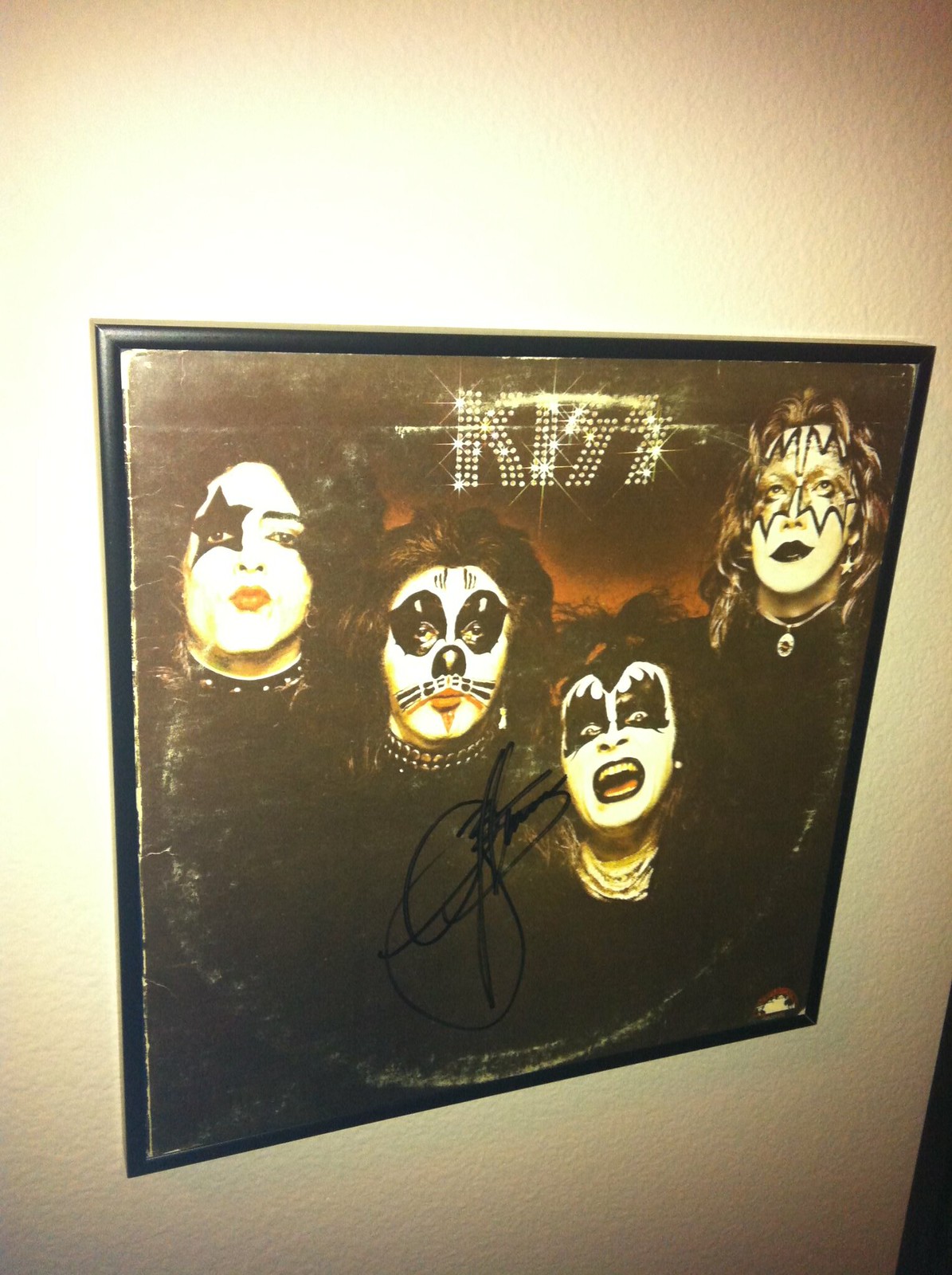The image is a tall, vertically oriented black-framed poster of the band KISS, mounted on a cream-colored wall. The iconic KISS logo at the top is emblazoned in sparkly diamond lettering. The poster features all four members of the band, each in their signature face paint and costumes. 

On the far left is Paul Stanley with his unmistakable white face makeup, red lips, and a black star over his right eye. His hair is black and curly. Next to him is the band member with cat-like face paint, featuring blackened eyes, a black nose, and drawn whiskers. He is also adorned with a spiked collar. In the center is Gene Simmons, identifiable by his menacing expression, white makeup, and the black flames painted around his eyes. He has his mouth open, adding to his fierce look. The final member on the far right has a lightning bolt design above his eyes, black lipstick, and long golden hair contrasting with the predominantly black hair of the other band members.

The poster is signed by the band members and there are hints of white distortion in a circular pattern, suggesting that the image could be from an album cover. The signature in the middle underscores its authenticity as a collectible item.